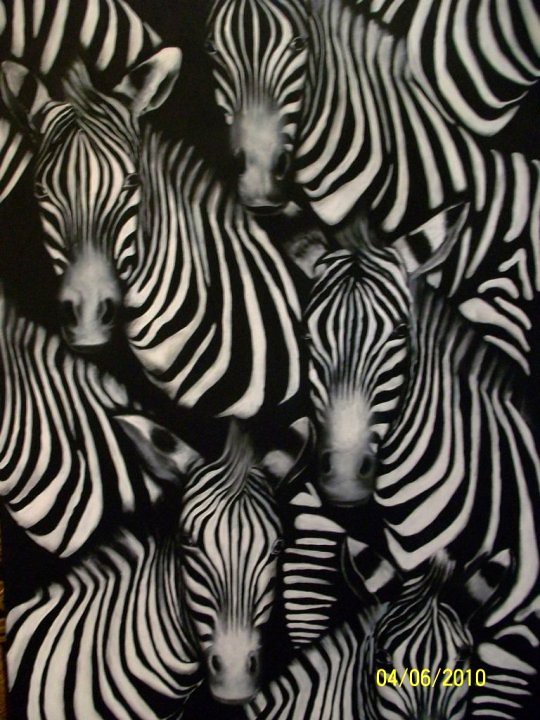This black and white manipulated photo, with a date stamp of 04-06-2010 in yellow text at the bottom right corner, features a highly detailed, distorted image of several zebras densely grouped together. The zebras' black and white stripes are prominently displayed, with variations from thin to thick patterns. Some zebras are staring directly at the camera with serious expressions, their large, gray noses, black nasal holes, and black slits for mouths standing out. Their spiked hair crowns their heads, and although their eyes are variably visible—some being prominent black ovals surrounded by little eyelids, others seeming almost non-existent—the overall effect is a surreal and somewhat out-of-focus depiction. The predominantly black background makes the manipulated, dream-like quality of the zebras' forms even more striking, amplifying the sense that they are merging into one another with blurred, indistinct features.